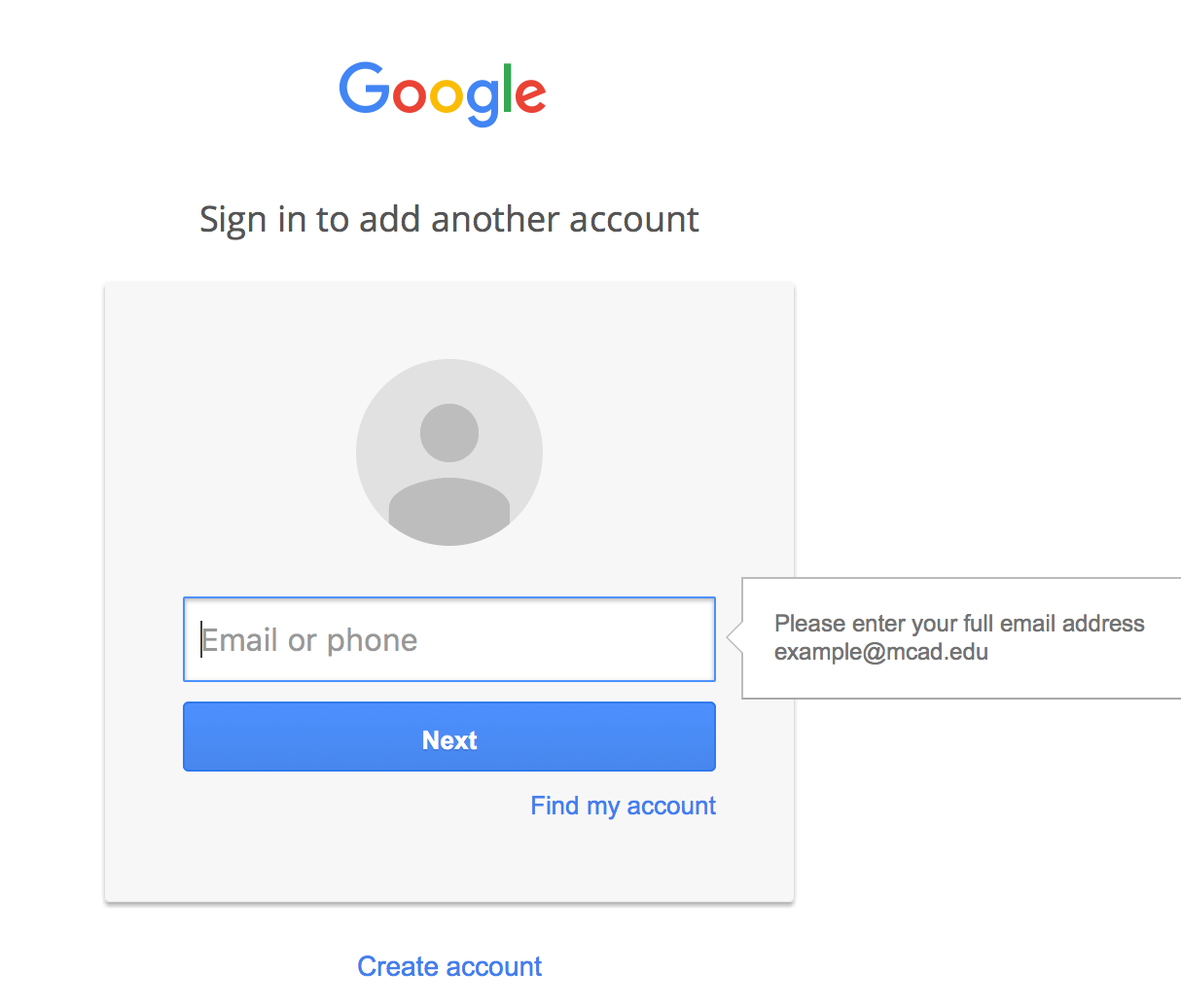The image is a screenshot of a Google login page. Positioned at the top left corner is the standard Google logo. Below the logo, in black text, it reads "Sign in to add another account." Beneath this text, there is a gray box displaying an empty profile picture placeholder.

Below the profile picture, there is a text field labeled "Email or phone." To the right of this text field, a small dialog box or reminder message appears, instructing the user to "Please enter your full email address." The reminder includes an example email format: "example@mcad.edu."

The layout is clean and minimalist, characteristic of Google’s design philosophy, emphasizing functionality and ease of use for its users.